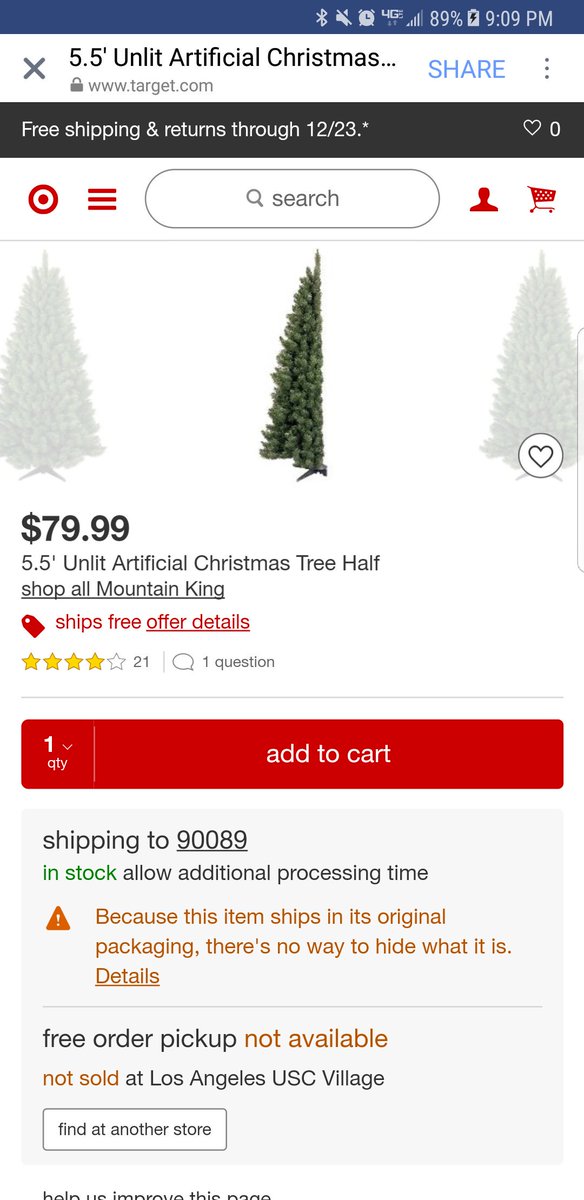The image depicts a shopping page from the Target website, specifically featuring an artificial Christmas tree. The URL displayed at the top is www.target.com. The central product is a 5.5-foot unlit artificial Christmas tree, presented with multiple angles showcasing both full and partial views. The tree appears slightly blurred in certain sections. 

The tree is priced at $79.99 and is sold by a seller named Mountain King. It is highlighted that the tree ships for free. The product has received an average rating of 4 out of 5 stars based on 21 reviews. There is one question about the item available on the site. 

The product page uses Target's signature red and white color scheme, and there is an option to add the tree to your cart. The item is currently available for shipping to zip code 90089, though additional processing time is required. 

A caution note at the bottom informs shoppers that the item ships in its original packaging and cannot be concealed, indicated by a yellow banner with an exclamation mark. The page also states that free order pickup is unavailable and that the tree is not sold at the Los Angeles USC Village location, though there is an option to check availability at other stores.

[Image: Target website product page showing a 5.5-foot unlit artificial Christmas tree for $79.99 sold by Mountain King, with free shipping. It has 4 out of 5 stars from 21 reviews, and is currently shipping to zip code 90089.]